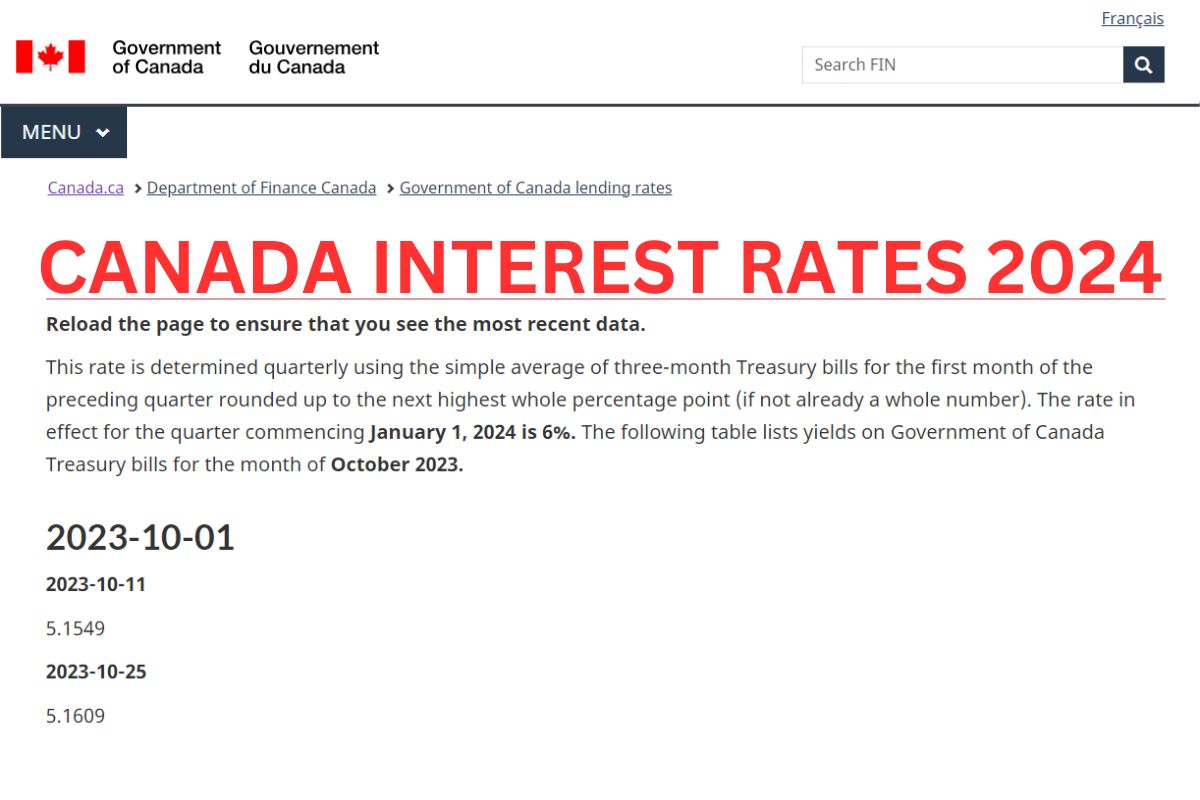**Screenshot of the Government of Canada Website on a Computer Monitor**

In this detailed screenshot of a Canadian government website displayed on a computer monitor, we see the official webpage for the Department of Finance Canada, specifically focusing on lending rates. 

**Top Section:**
- **Icon and Title**: The upper left corner features a Canadian flag icon accompanied by the text "Government of Canada," which is also presented in French as "Gouvernement du Canada."
- **Search Bar**: To the right, there's a search bar with the text "search, F-I-N" and a white magnifying glass icon inside a black square.
- **Language Option**: Above the search bar, "Francais" is underlined, indicating that users can switch to the French version of the website.

**Navigation and Menu:**
- **Menu Button**: Directly beneath a dark grey line that spans the width of the screen, there is a black rectangle labeled "menu" in white letters, along with a white downward arrow suggesting a dropdown menu.
- **Breadcrumb Navigation**: Below the menu, a breadcrumb trail shows "Canada.ca" > "Department of Finance Canada" > "Government of Canada Lending Rates," indicating the webpage's navigation path. Each segment is clickable to take the user to the respective sections.

**Main Content:**
- **Header**: In large, bold red capital letters, the main header reads "Canada Interest Rates 2024."
- **Update Notice**: Following the header, a notice in black text advises users to reload the page to see the most recent data.
- **Rate Determination Explanation**: An explanatory paragraph in black text describes how the rate is determined quarterly: "This rate is determined quarterly using the simple average of three month treasury bills for the first month of the preceding quarter, rounded up to the next highest whole percentage point (if not already a whole number)."
- **Current Rate**: Highlighted in bold, the current rate for the quarter commencing January 1, 2024, is listed as 6%.

**Interest Rate Table:**
- **Table Header**: A table beneath the explanatory paragraph provides the yields on Government of Canada treasury bills for October 2023, with "October 2023" in bold for emphasis.
- **Data Entries**: The table includes dates formatted as "2023-10-01" and "2023-10-11." Corresponding to these dates are the interest rates: 5.1549% on October 1, 2023, and 5.1609% on October 25, 2023, indicating a slight increase in the rates over the month.

This comprehensive view provides users with essential information about lending rates, including how they are calculated and recent figures, ensuring transparency and accessibility on the Government of Canada's financial policies.